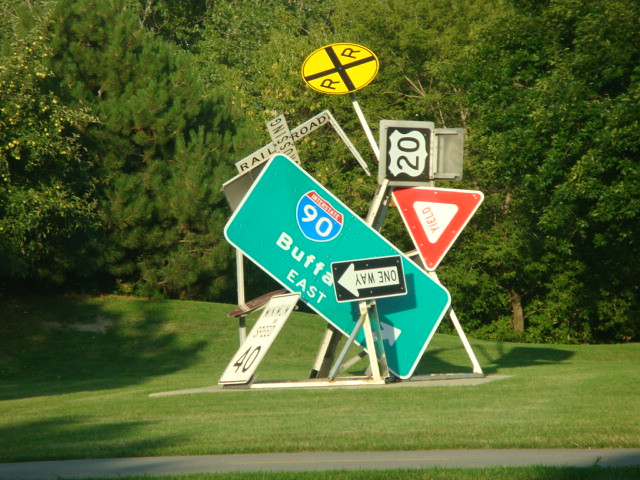The image showcases a cluttered assortment of various road signs situated near a dense wooded area with numerous tall trees. The foreground features a neatly trimmed, golf-course-like short grass. Among the signs, a prominent Interstate 90 sign visibly stands out, displaying directions towards Buffalo and the East with an arrow pointing to the right. In front of it, an upside-down one-way sign adds to the chaotic arrangement. Additionally, a tilted, triangular yield sign with a red border and white center, bearing the word "YIELD" in bold red letters, is also noticeable. The signs are haphazardly grouped together, with some leaning against or falling onto others, creating a scene of disarray.